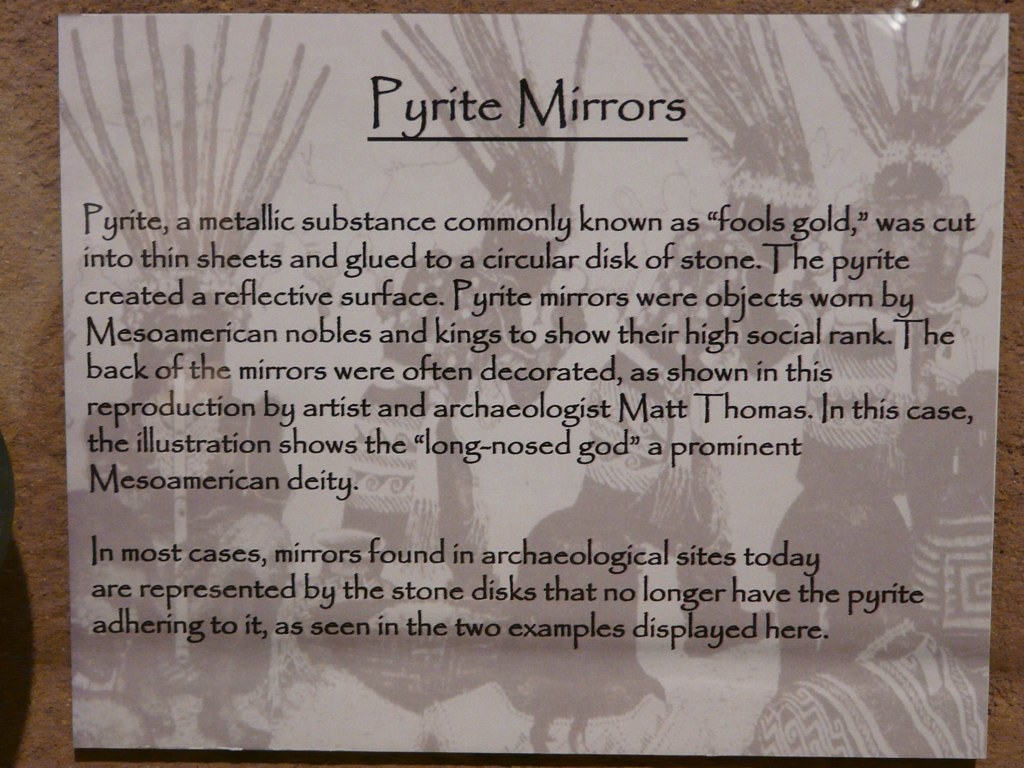This image captures a detailed display card from a museum showcasing information on Pyrite mirrors. The card, printed on a gray or white sheet of paper with black text, is set against a background that appears to be made of marble with faintly visible figures in traditional cultural dress, possibly Native Indian dancers, rendered in sepia tones of gray, brown, and white. The text on the card is headed with "Pyrite Mirrors" underlined with a black line, followed by an informative description. 

It reads:

"Pyrite, a metallic substance commonly known as 'fool's gold,' was cut into thin sheets and glued to a circular disk of stone, creating a reflective surface. Pyrite mirrors were objects worn by Mesoamerican nobles and kings to show their high social rank. The back of the mirrors were often decorated, as shown in this reproduction by artist and archaeologist Matt Thomas. In this case, the illustration depicts the 'long-nosed god,' a prominent Mesoamerican deity. In most cases, mirrors found in archaeological sites today are represented by the stone disks that no longer have the pyrite adhering to them, as seen in the two examples displayed here."

This descriptive card not only informs visitors about the historical and cultural significance of pyrite mirrors but also showcases a beautifully detailed reproduction of these artifacts.